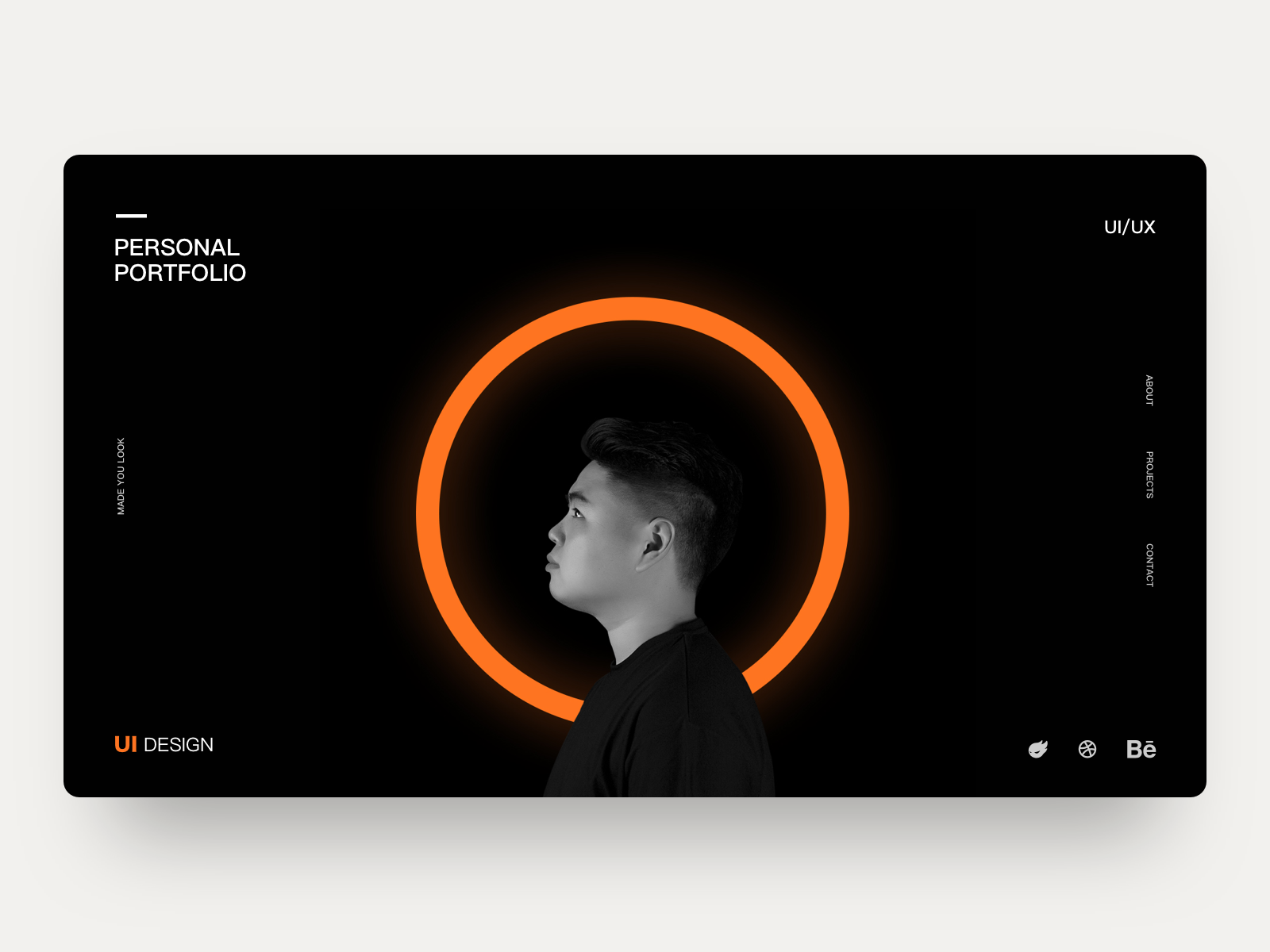This image depicts a section of a website designed as a sleek, minimalist business card. The background is a light gray color, which enhances the central black business card-shaped element. In the middle of the card, there is a photograph of a man facing left. He has black hair, a clean-shaven face, and is wearing a black T-shirt. Behind him, an orange circle adds a pop of color to the monochromatic theme.

In the upper left corner of the card, there's a stylized icon composed of a line and a short line. Beneath this icon, in white text, it reads, "Personal Portfolio." Along the center of the left side, more white text is visible. In the bottom left corner, there is an orange "UI" followed by "design" in white text.

On the upper right corner, "UI/UX" is written in white text. The right side of the card lists “About,” “Products,” and “Connect” in white text. In the bottom right corner, there are several white icons, though their specific design is not detailed. This organized and visually appealing layout highlights key information and contact options effectively.